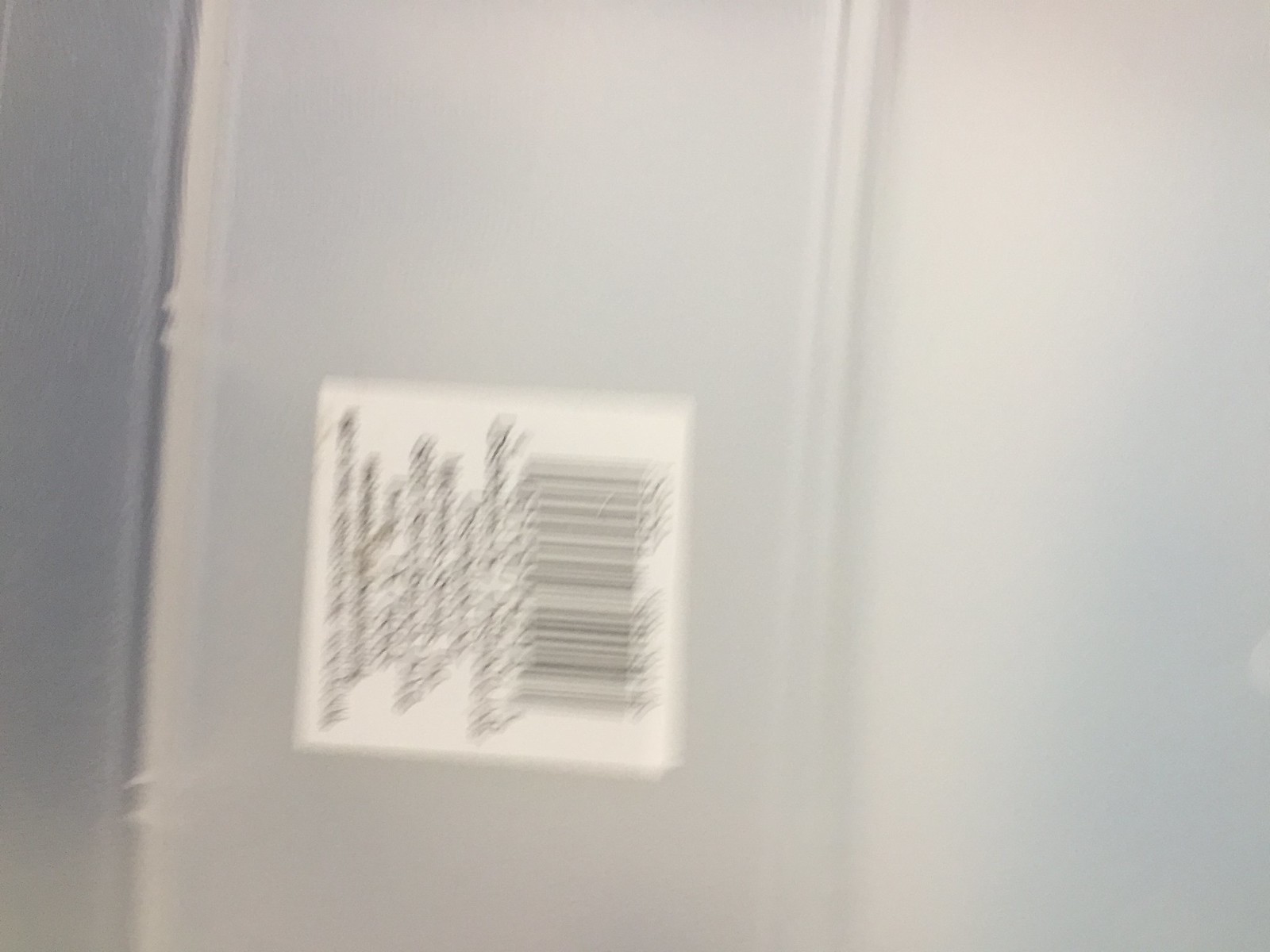The photograph captures a blurry, low-quality, landscape-oriented image focusing on a white sticker positioned on the middle section of a silver metal background. The sticker contains a barcode with several lines of illegible black text beneath it, all oriented vertically. The metal background features varying shades of gray, with a distinct dark gray area on the far left and lighter gray panels transitioning toward the right. These panels are separated by vertical ridges, creating a concave and convex appearance. The overall effect is marred by significant motion blur, obscuring finer details across the entire image.